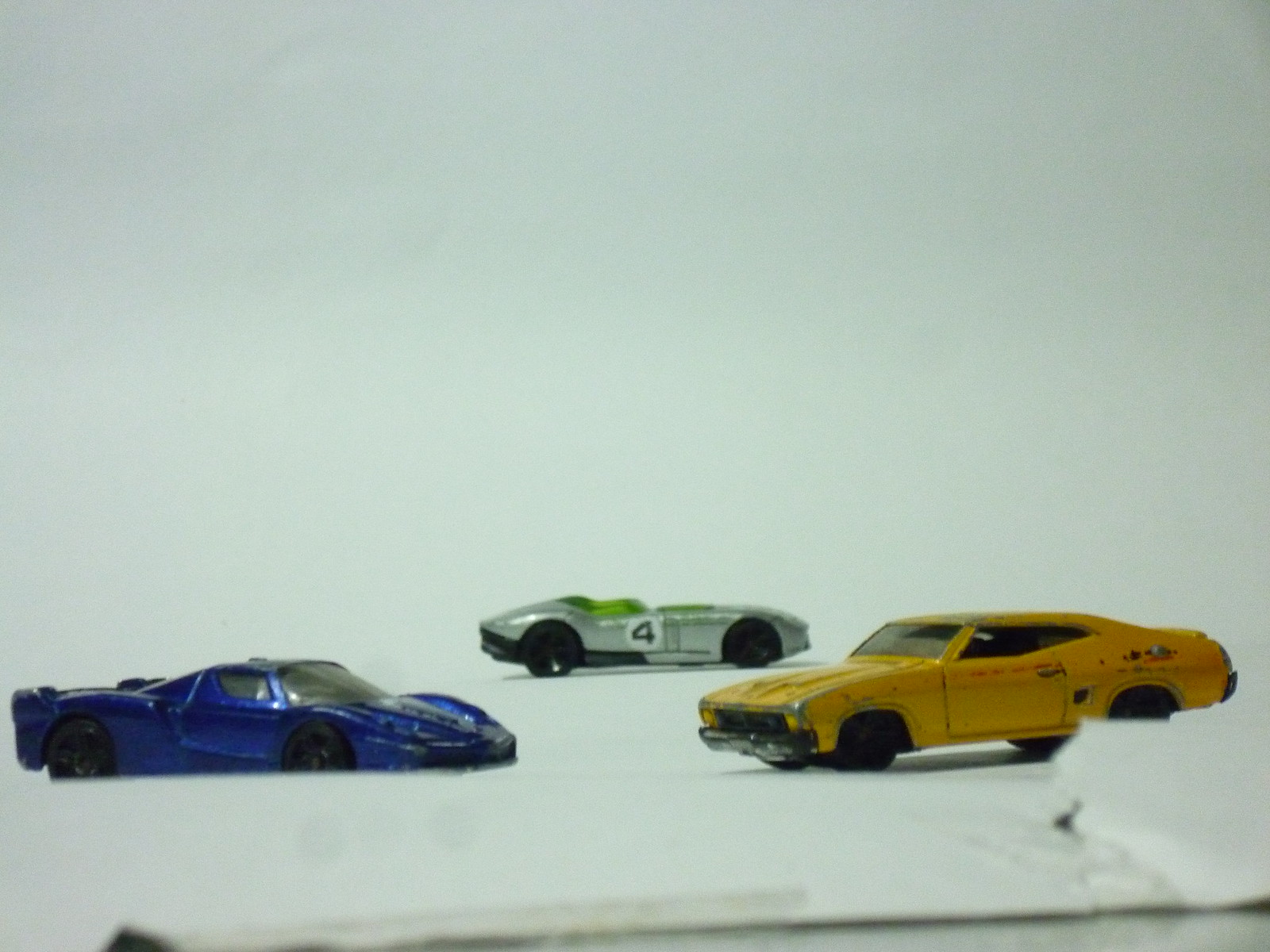This image showcases a close-up view of three Matchbox cars aligned on a white surface with a seamless white background. To the left, a deep blue, low-profile sports car, resembling a Lamborghini, is positioned at an angle, allowing a glimpse of both its front and side, while its tail is oriented to the left. This car features a distinctive spoiler and black tires. On the right, there is a mustard-yellow old-time muscle car with visible dings and scratches. It is angled such that its front faces left with its tail directed to the right. This yellow car also sports red markings and black tires. Positioned between them, and slightly to the rear, is a sleek silver European race car, identifiable by its green interior and convertible design. It has a white circle with the number 4 emblazoned on its door and is oriented towards the right of the photo. All three cars are framed against the pristine white backdrop, highlighting their vibrant colors and distinctive characteristics.